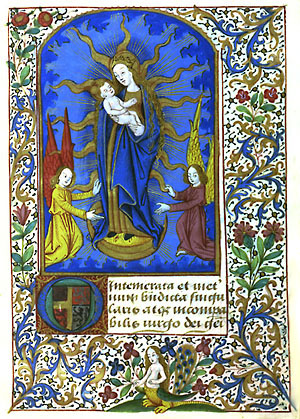The image is a vibrant piece that resembles a religious print, possibly of the Virgin Mary holding a porcelain-colored baby. The central figure, located towards the upper left, is backed by a rich blue background with a gold edge. She is adorned in a long blue robe with gold accents and features long, flowing gold filigree strokes extending outward like rays. The background of the image is ornate and highly colorful, filled with elegant, curving brush strokes and flowers.

Flanking the central figure are two kneeling women, who may represent angels. The one on the left is dressed in a yellow long-sleeve dress and has red wings, while the one on the right is in a burgundy long-sleeve dress with gold wings. Both appear to be attending to the central figure's robe. Below this tableau, there is a family crest and a cursive inscription in Latin or another non-English language.